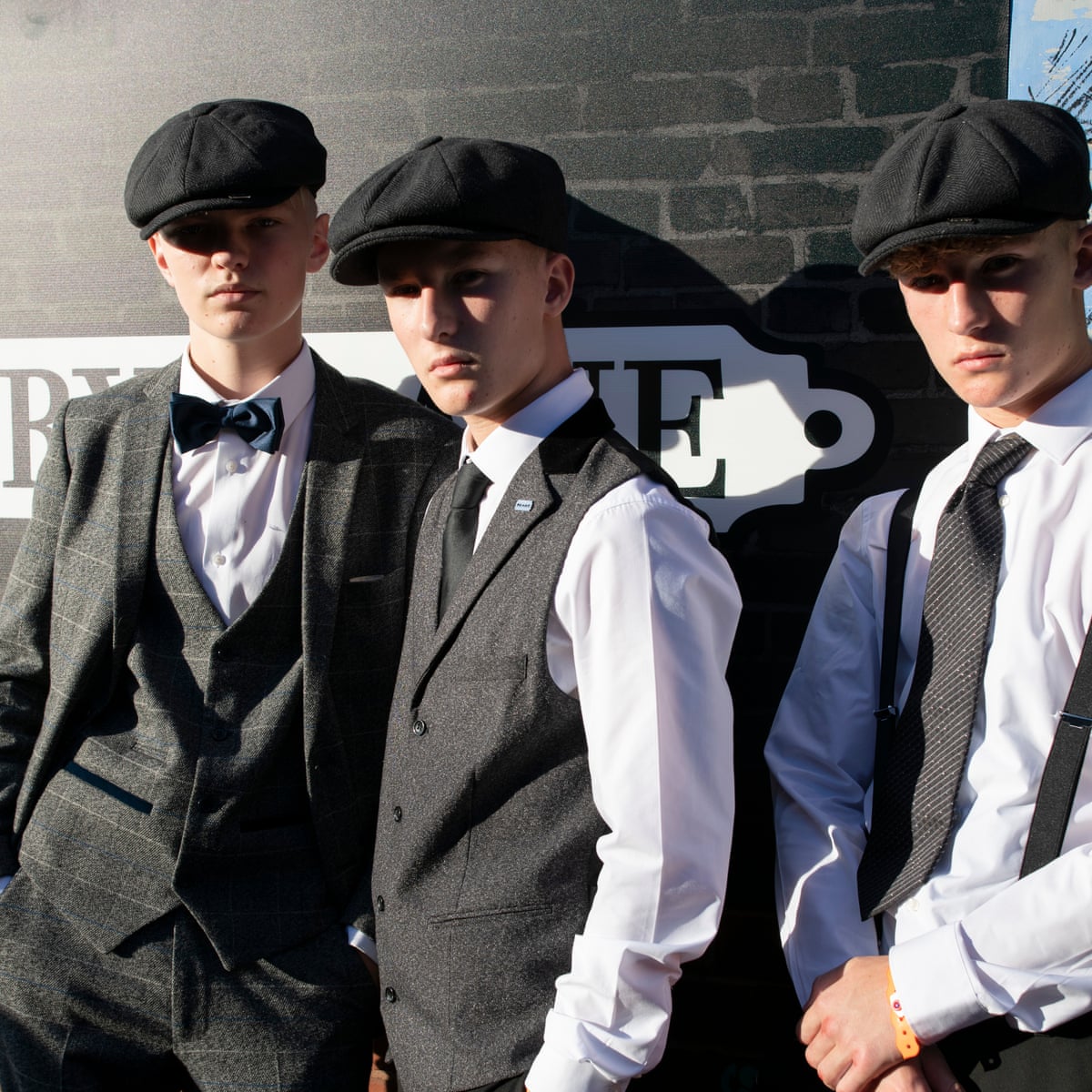The photograph captures three young men posing elegantly in front of a gray brick wall, all looking directly at the camera with neutral expressions. Each is adorned in a black newsboy cap, adding a sense of uniformity among them. The young man on the left is dressed in a gray three-piece suit, complete with a white shirt and a black bow tie, enhancing his sophisticated appearance. The man in the center, slightly turned away yet facing the camera, stands out with his gray-black vest worn over a crisp white shirt, reminiscent of a traditional suit minus the jacket. Finally, the young man on the right, with arms crossed and holding his wrist, sports a similar crisp white shirt paired with suspenders, foregoing a jacket but maintaining a polished look. Together, they present a harmonious yet individually distinguished style against the backdrop of the brick building.